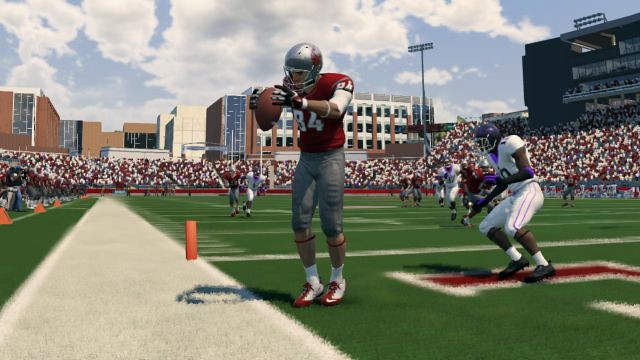The image appears to be a highly realistic digital rendering, resembling a screenshot from a video game or an AI-generated scene. It portrays a vibrant moment in a football stadium. In the upper background, a clear blue sky adorned with fluffy white clouds sets an idyllic atmosphere. Below, a sprawling array of brick buildings with a brown hue suggests a college campus setting.

The crowd, represented by colored dots, fills the stands in a U-shape around the field, creating a bustling, lively scene. The football field features bright green artificial turf with crisp white borders. In the foreground, two football players dominate the scene. The primary player, seemingly in mid-action capturing the ball, sports a maroon jersey with either the number 34 or 84, gray pants, and white shoes with red laces. His silver helmet gleams under the stadium lights as he grasps a brown football. 

Nearby, an opposing player dressed in a white uniform with a purple helmet adds to the competitive tension of the moment. The grandstands in the distance are filled with spectators in white and red, adding a wave of color and excitement to the scene.